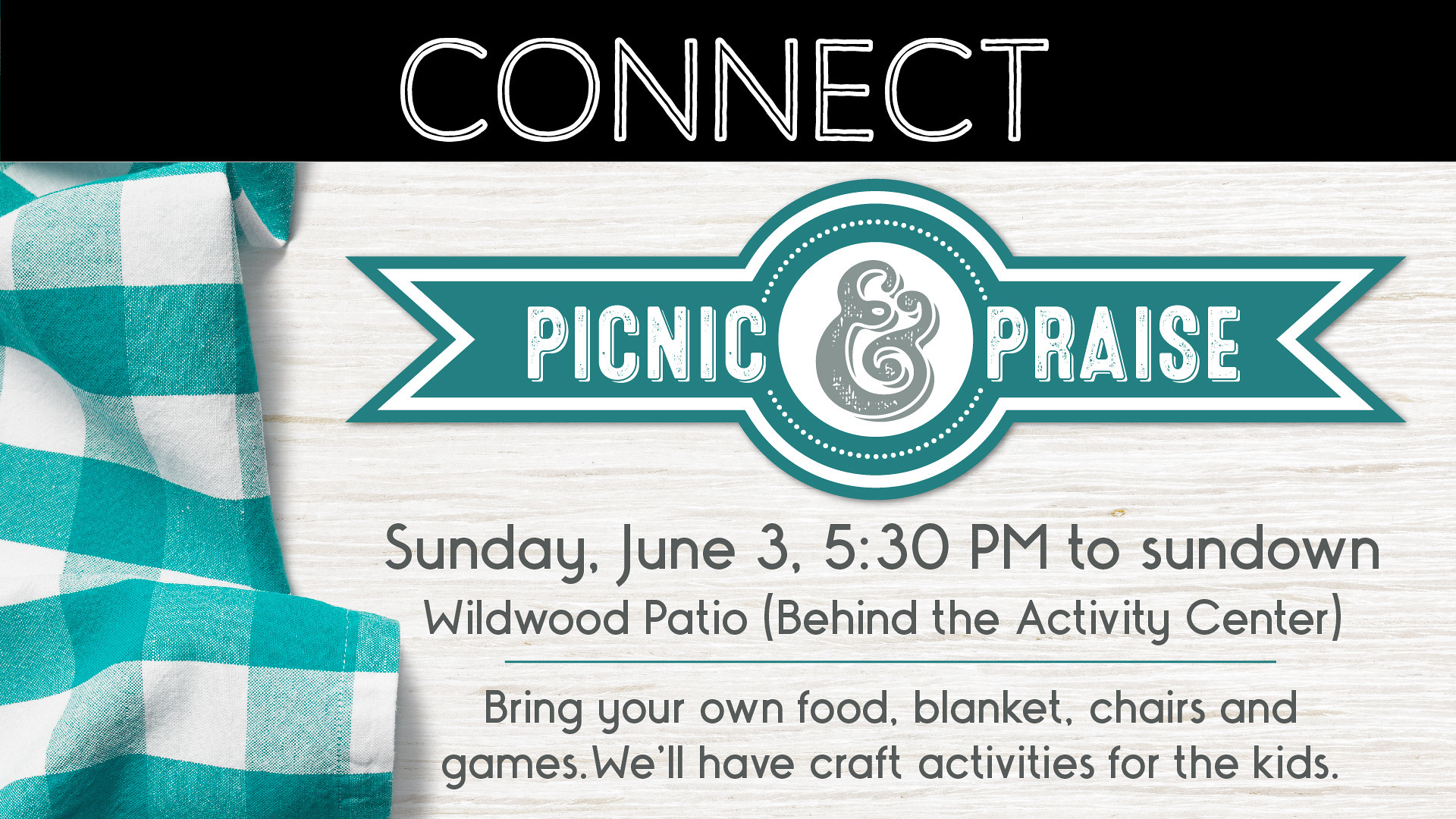This image is a digital advertisement with a white and wooden design background, featuring a detailed layout and a picnic theme. At the top of the advertisement, there's a black bar with the text "Connect" written in white letters. Below, in a ribbon-shaped design, it reads "Picnic & Praise" with "Picnic" on the left side, "Praise" on the right, and an ampersand in the middle. The event details state, "Sunday, June 3rd, 5:30 p.m. to sundown," happening at the "Wildwood Patio, behind the activity center." The ad also mentions to "Bring your own food, blanket, chairs, and games," and highlights that "craft activities for the kids" will be provided. On the left-hand corner, there's a blue and white checkered picnic blanket or tablecloth, adding to the picnic theme. The primary colors involved are white, black, teal, and gray, and the overall design gives a warm, inviting feel suitable for a family picnic event.